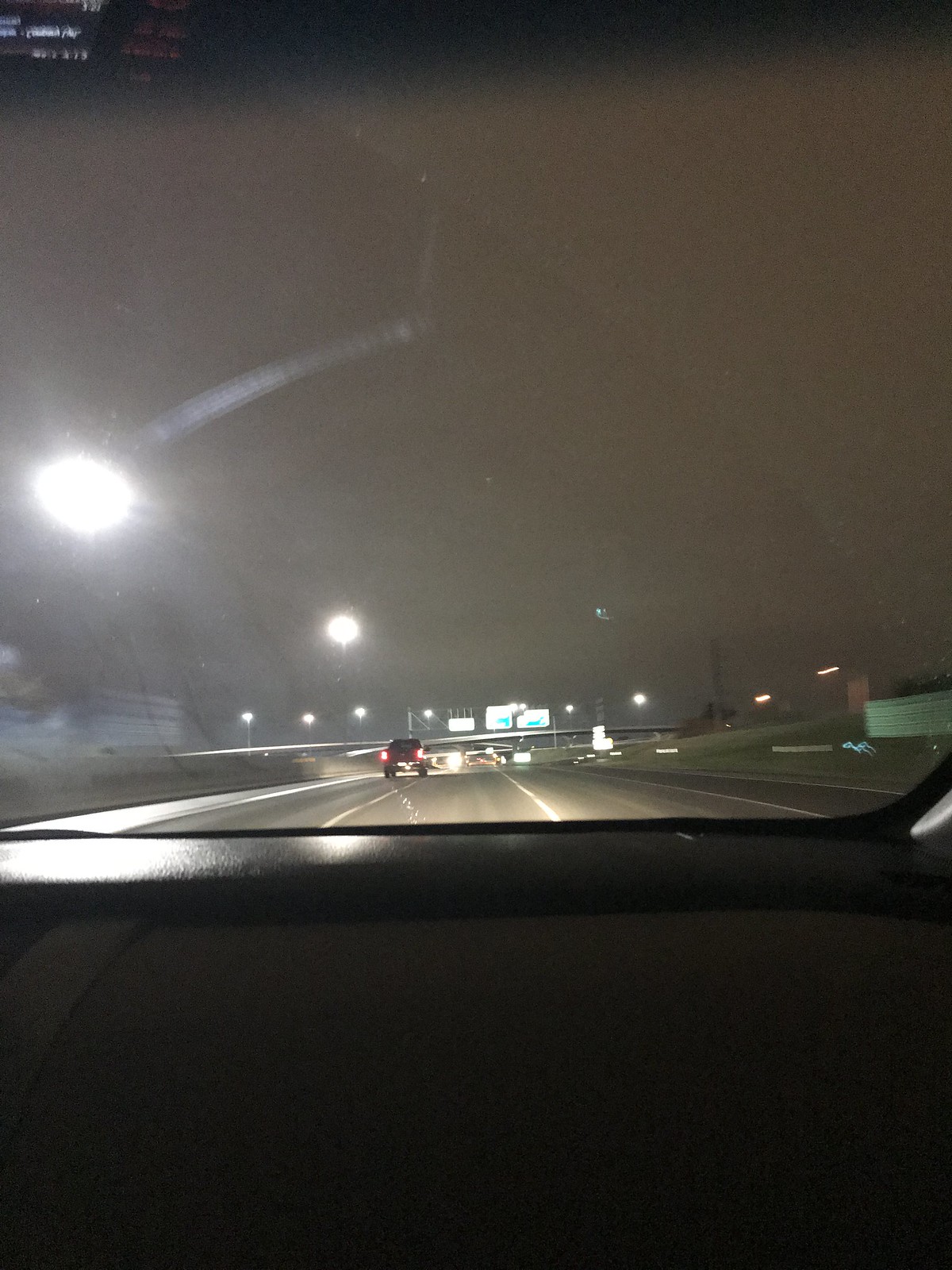This nighttime photograph is taken from the passenger seat of a moving car on a four-lane road. The scene is viewed through the car’s front windshield, with the black dashboard partially visible below. The car is traveling on the right side of the two left lanes, and the road features a bridge overpass visible ahead. Street lamps illuminate the scene, and a truck is seen driving in the lane just ahead, its taillights glowing in the darkness. 

Reflective green freeway signs and the well-lit overpass add to the brightness despite the nighttime setting. The sky appears grey, possibly due to ambient city lights. The road is flanked by upward grassy slopes on both sides, with structures like buildings or walls visible on the left side slope. Additionally, the reflection of the car’s console and the camera flash can be seen on the windshield, adding to the sense of motion and capturing the interior's dimly lit atmosphere.